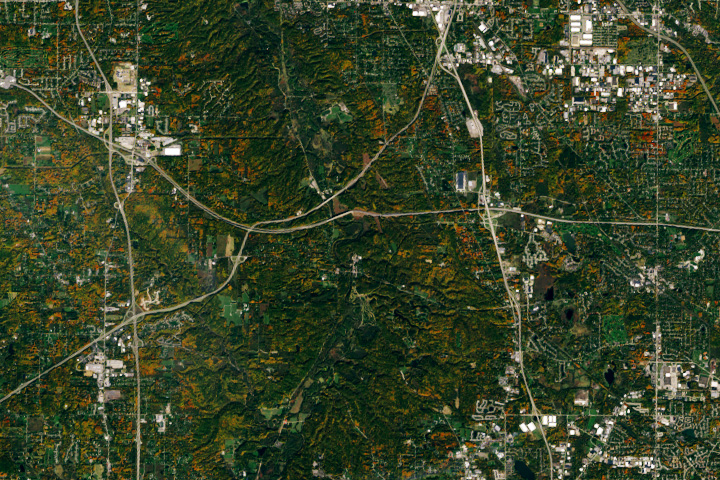This highly detailed, full-color aerial photograph, possibly a satellite image, provides a comprehensive view of a landscape composed of both human settlements and natural wilderness. The image itself is square and captures an expansive view from a very high altitude, offering a broad perspective of the terrain below. The photograph showcases four clusters of human activity—each situated in a different corner of the image (upper left, upper right, lower left, and lower right). These urban centers consist of numerous white buildings, indicating populated areas, yet specific details of the structures are not discernible due to the high altitude of the shot.

Connecting these urban clusters are thin, squiggly gray lines representing roads and highways. These roads meander through a predominantly green landscape, interspersed with patches of yellow, orange, and brown hues, suggesting that the photograph was taken during early fall when the foliage is transitioning colors. Additionally, several lakes are visible in the lower right portion of the image, providing a contrasting element to the surrounding terrain.

One notable feature is a raised, elevated area in the middle of the image, which appears to be a mountainous region or a significant topographical elevation running vertically across the center. This distinct element further enhances the depth and complexity of the landmass depicted in the photograph. Overall, the image offers a rich, multifaceted view of an intricate blend of urban and natural elements.